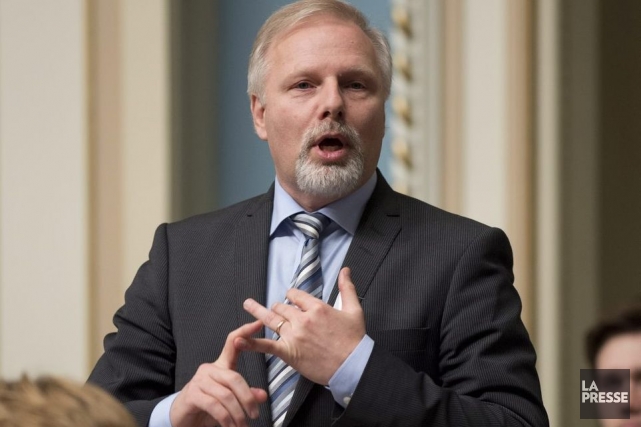A man with a gray goatee and short gray hair is seen placing the index finger of his right hand on the pinky finger of his left hand. His mouth is open as if he is mid-sentence or exclaiming something. He is dressed in a black suit over a blue undershirt, complemented by a white and gray striped tie. In the bottom right corner of the image, the text "La Presse" is visible. The background features a white wall, a blue doorway, and a white and gold spiraled pillar. To the right of the man, another person with short black hair can be seen. In the front left part of the scene, the top of another individual's head is visible, with gold or yellow hair. The setting seems formal, perhaps an indoor public or official venue.